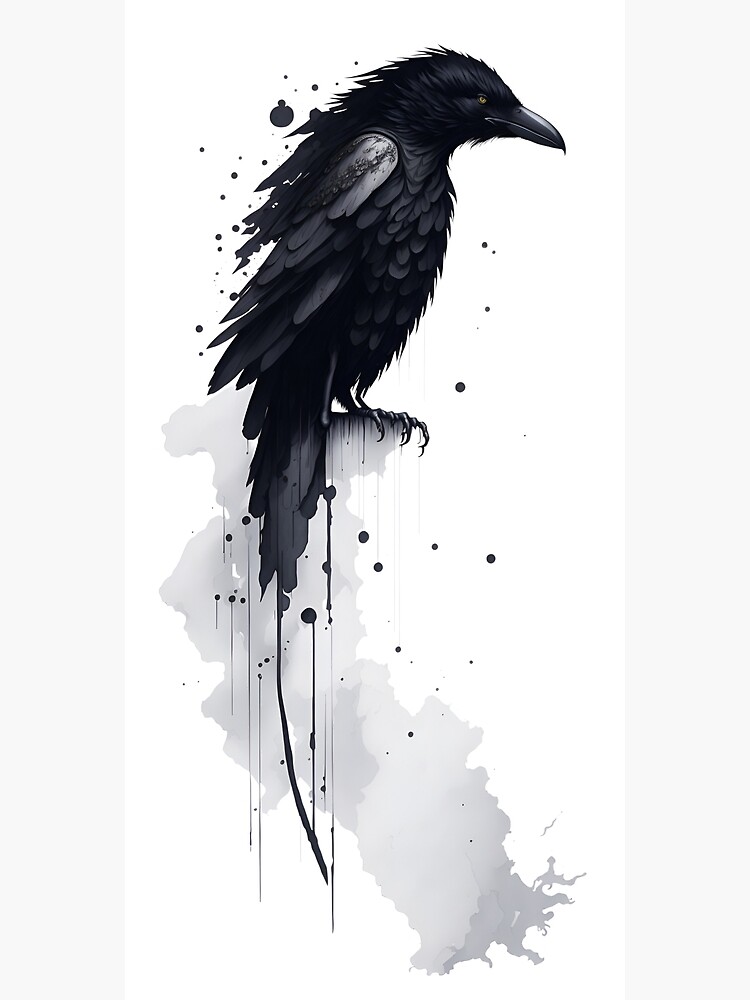This detailed illustration features a raven depicted in watercolor, perched on a diffuse, gray splotch suggestive of either a cloud or a cliff. The raven, portrayed in an intense side profile facing right, showcases ruffled, black feathers and a striking yellow eye that conveys a sense of upset or intensity. Black paint drips around the raven add a dynamic quality, cascading down the white background of the painting. The surrounding area remains minimalistic, highlighting the raven's stark black figure and the grayish spot it rests upon. Borders of a slightly darker gray frame the white background on two sides, emphasizing the central focus on the compelling, enigmatic raven.